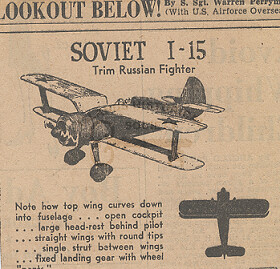This photograph captures a yellowed newspaper article titled "Look Out Below" by Staff Sergeant Warren Ferry, under the oversight of the US Air Force. The central feature of the article is a detailed drawing of a Soviet I-15 Russian fighter airplane, accompanied by annotations describing its features. The image showcases an old-time military prop plane with stars on its wings, an open cockpit, a large headrest behind the pilot, straight wings with rounded tips, a single strut between the wings, and fixed landing gear with wheels. Below the main drawing, there's a note emphasizing, “note how top wing curves down into fuselage.” In the lower right corner, the article includes an additional view of the aircraft from above, highlighting its distinct design. The article is from the World War II era, reflecting historical military aviation commentary.